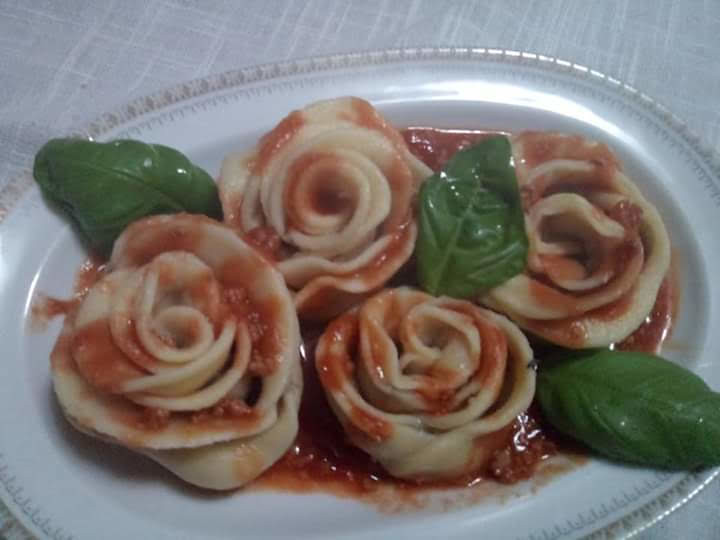This photograph, presented in landscape orientation, captures a meticulously styled culinary presentation. The centerpiece is an oval-shaped, shallow white ceramic dish with a cream-colored fluted edge, placed on a textured grey tablecloth. Inside the dish, four rose-shaped pasta creations, off-white in color, are beautifully arranged. Each rose is intricately fashioned from flat dough, giving a realistic floral appearance. A vibrant red tomato sauce generously covers the pasta roses, pooling slightly at the bottom of the dish. Nestled among the roses are three fresh green basil leaves, strategically placed—one at the top left, one at the top right, and one at the bottom right—adding a touch of color contrast and garnish. The photograph, though slightly blurry, vividly captures the essence of representational realism in food photography.